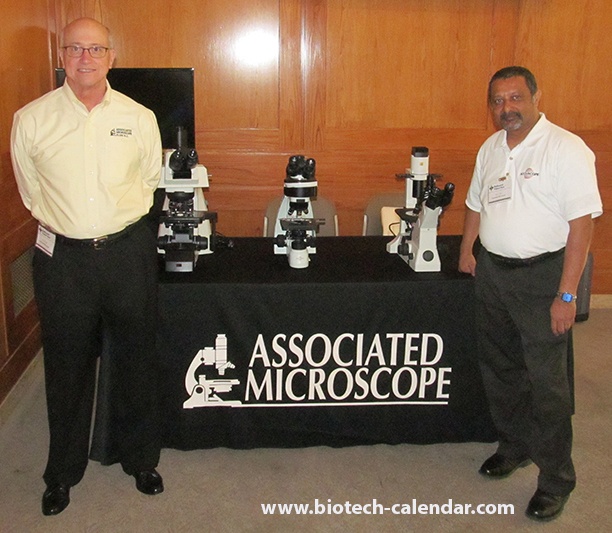The image shows two middle-aged men standing in front of a table covered with a black tablecloth. The tablecloth features white text that reads "associated microscope" alongside the white outline of a microscope. The men are positioned against a backdrop of large wooden paneling, hinting at an indoor setting that could be an office or a trade show.

The man on the left is taller, Caucasian, and slightly bald, wearing black shoes, black pants, and a long-sleeved yellow button-down shirt with a collar. He also has glasses and his name tag is clipped to his belt. The man on the right is shorter, with a tan complexion, likely Hispanic, sporting black shoes, black pants, and a collared white polo shirt. He also has dark hair, a mustache, and a goatee. His name tag is attached to his shirt, and he wears a watch with a blue face.

On the table between them are three microscopes, each featuring a white base and black details. In the lower right corner of the image, there is a watermark with the URL "www.biotech-calendar.com," adding a professional touch to the setup.